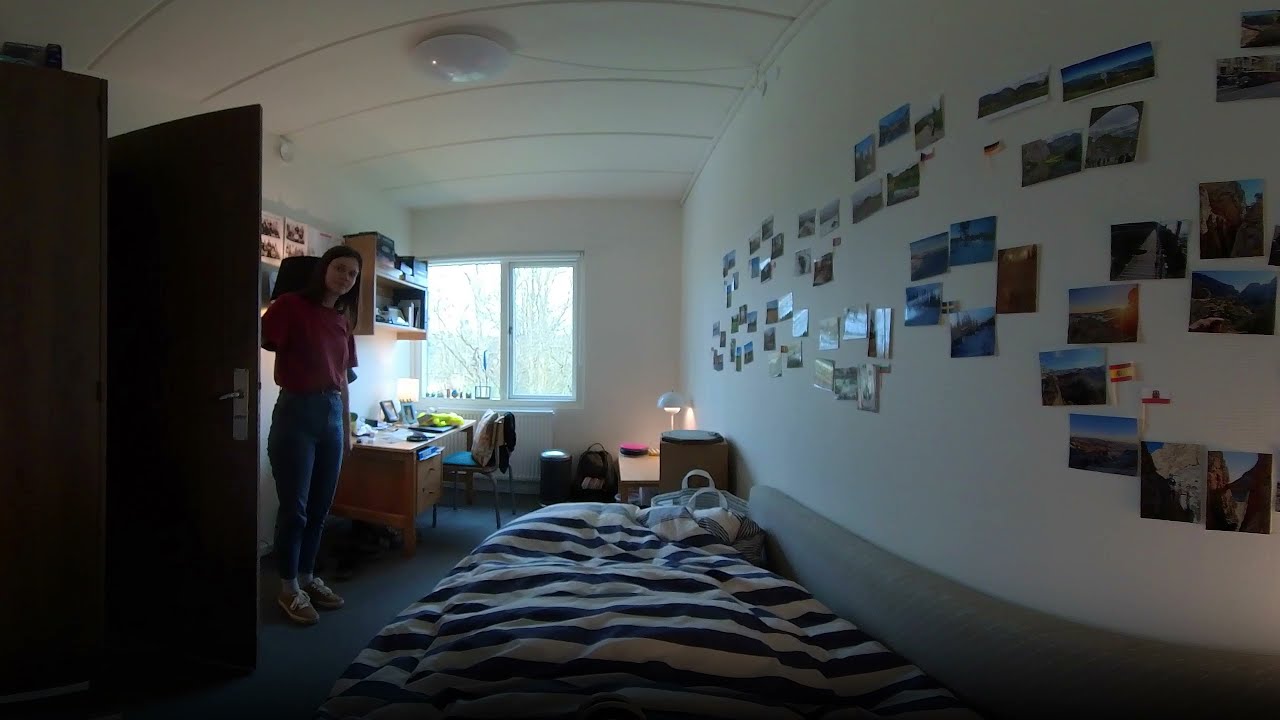This image depicts a college dorm room taken with a fisheye perspective, showing a neat and personalized living space. Central to the photograph is a young Caucasian woman with straight brown hair, dressed in a red short-sleeved t-shirt tucked into blue jeans and wearing gray or tan sneakers with gray socks. She is standing near the open wooden door, partially obstructing her right arm. 

The room features white walls heavily decorated with numerous photos and postcards. A blue and white striped bedspread covers a futon or bed situated along the left wall. Nearby, a wooden desk is positioned in the corner, adorned with various implements and a lamp. Above the desk, a shelf holds an assortment of books and papers. In front of the desk is a chair with a pillow placed on it.

Further details include a window at the end of the room that brings in daylight, framed by a simple white frame, and a glimpsed tree outside. Ornaments are arranged on the windowsill, adding a touch of personalization. In front of the bed, there’s a striped blue and white bag on the floor. The ceiling is white, with a light fixture in its center, enhancing the bright and organized atmosphere of the room.